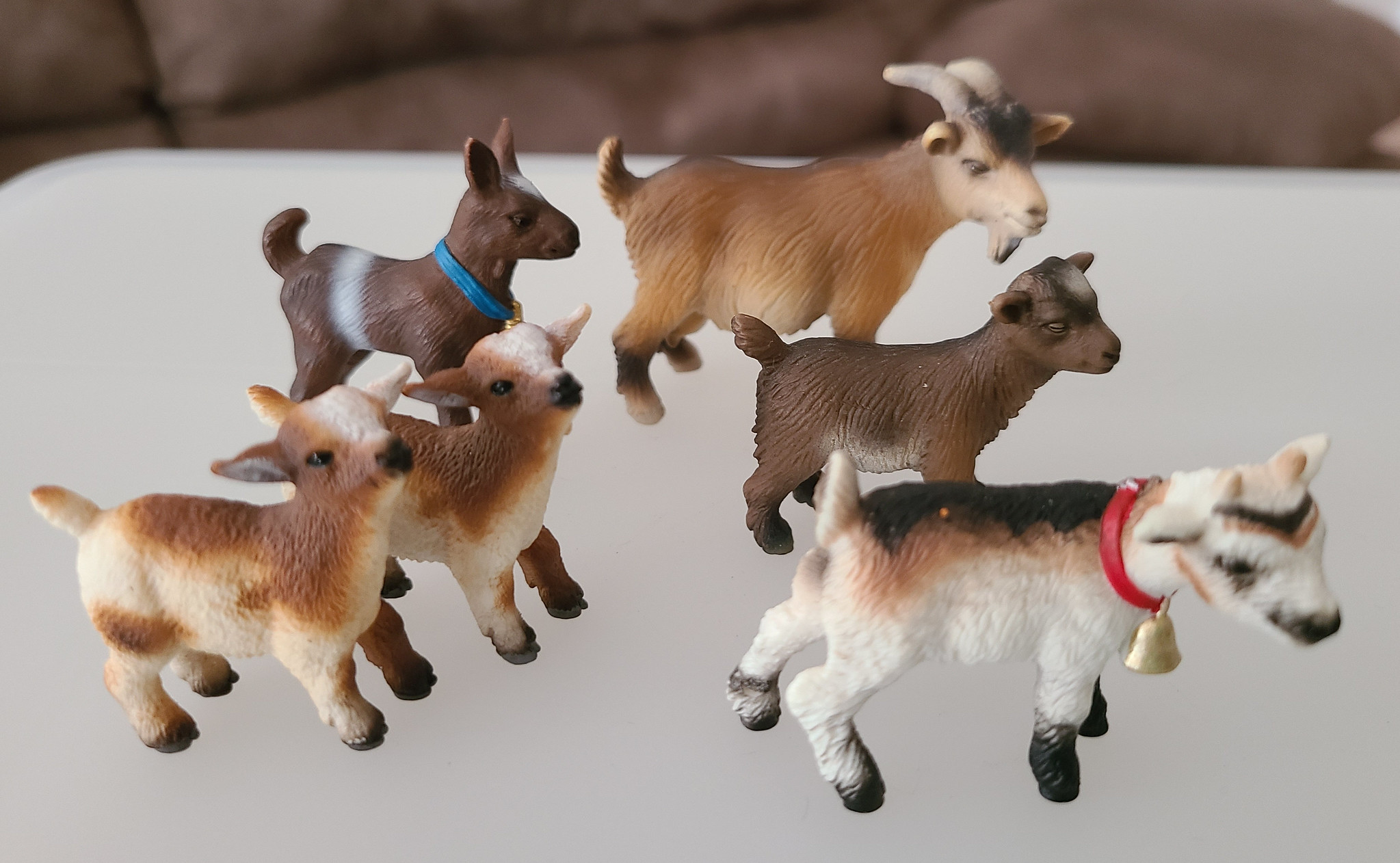In this photograph, six realistic-looking, molded plastic farm animals are meticulously arranged in two columns on a semi-transparent coffee table with a white top, set against the backdrop of an out-of-focus couch with padded backrest and armrest. In the foreground stands a white cow with black markings, sporting a red collar with a bell and two horns. To the cow's right, there is a dark brown sheep and a large tan billy goat with prominent curved horns. Two identical, baby-like sheep with black noses, tan backs, and black eyes stand to the left, while another sheep, characterized by black and white patches including a black back and tan belly, completes the scene. In the background, a brown dog with a lighter stripe around the belly and a collar with a name tag adds an additional layer of depth to this quaint rural display.